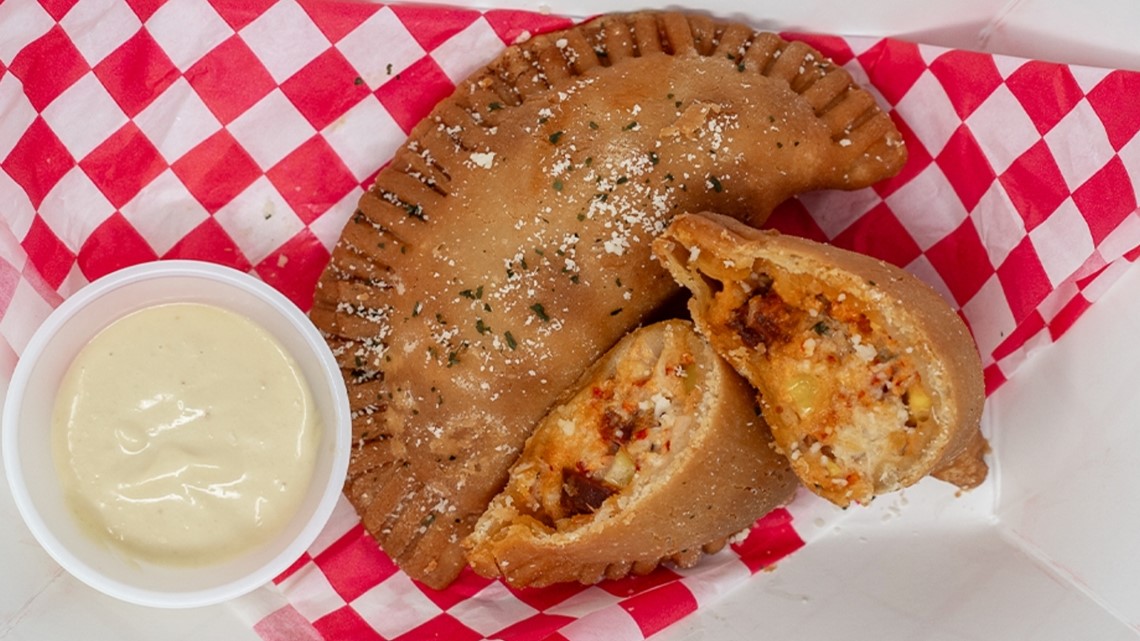The image depicts a crescent-shaped pastry, closely resembling a calzone or a similar stuffed bread, placed diagonally from the top to the bottom of the frame. It rests on a red and white checkered napkin. The golden-brown pastry, which appears to have been baked to a crisp, features indentations along the edge, likely made with a fork to seal the dough. The outer surface is dusted with a white powder, possibly Parmesan cheese, and garnished with green herbs. The pastry is partially cut open, showcasing a savory filling of eggs, bacon, cheese, tomatoes, and onions, with hints of a creamy white sauce inside. Additionally, in the lower left corner of the image, there is a small white plastic container holding a thick, glossy white condiment, which might be sour cream. The entire scene is set within a box, evident from the view in the lower right corner.